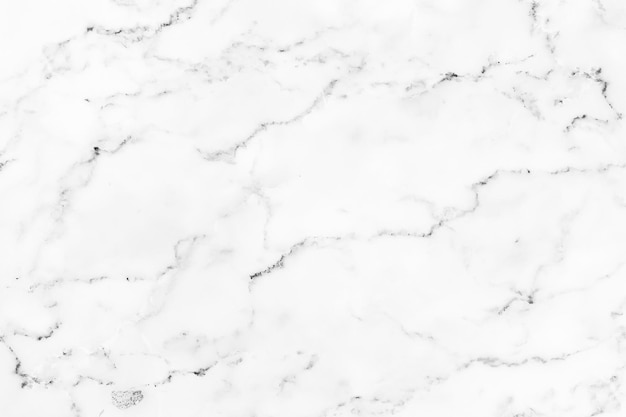This image is a horizontally aligned rectangular photograph without any borders or text. It depicts a marble surface featuring a predominantly white stone substrate with irregular black veins criss-crossing throughout. The white areas are more prominent in the center of the image, giving the impression of larger patches of white with crooked black lines, while the corners display smaller, more intricate patterns of black outlines. The marble surface could be part of a countertop or a wall slab, and the lack of surrounding context or additional color emphasizes the intricate and natural patterning of the black veins against the white stone. The image appears as though it could serve as a promotional visual showcasing the aesthetic details of this marble material.